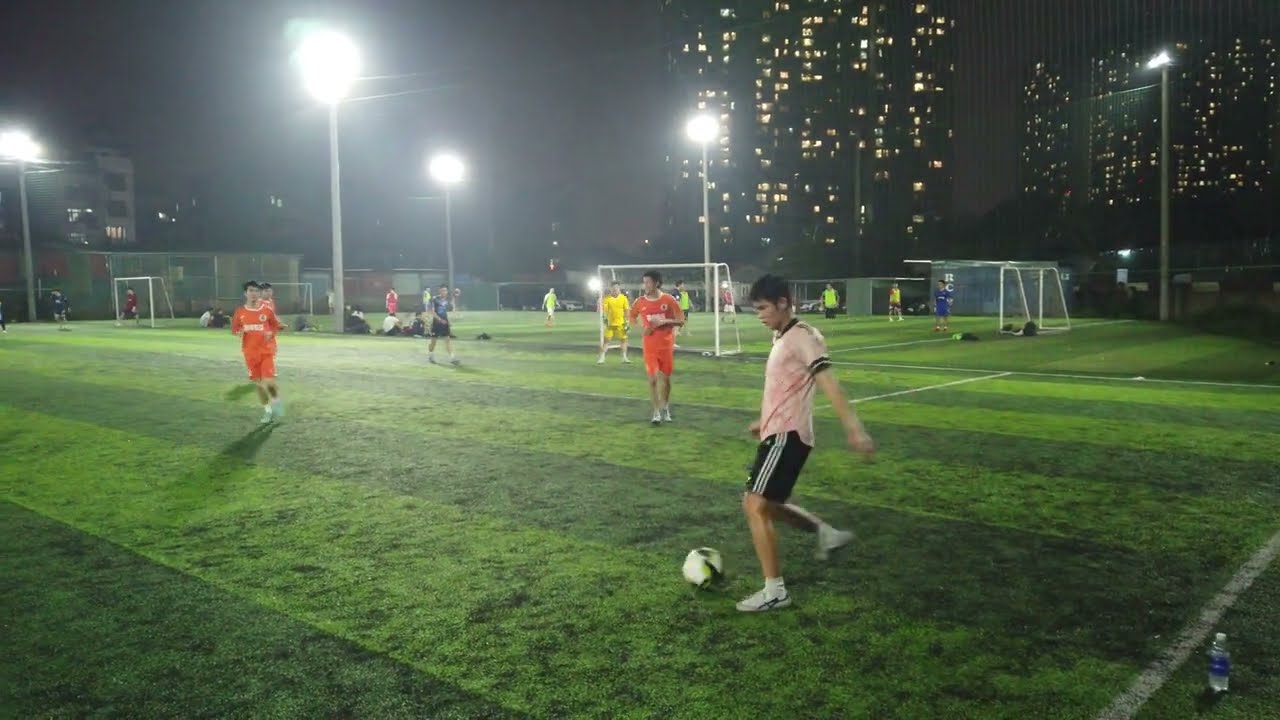This detailed, nighttime photograph captures a vibrant soccer scene in what appears to be a bustling metropolitan area, characterized by towering high-rise buildings with their windows glowing against the dark sky. The field, which is a high-quality artificial turf marked with a straight pattern, is illuminated by various lamps and poles. The scene shows multiple soccer games or practices occurring simultaneously, evidenced by the numerous soccer nets scattered across the field. In the forefront, a man with dark hair, wearing a pinkish-white shirt, black shorts with white stripes, and white shoes, is captured mid-kick, intensely focused on the soccer ball at his feet. Behind him, three players in orange jerseys with white shoes are approaching, adding to the dynamic atmosphere of the image. More players in varied colored uniforms — red, yellow, green, blue, and gray — are seen scattered across the field, emphasizing the diversity of teams practicing. The photograph, with its realistic and representational style, offers an eye-level view that draws the viewer into the spirited and energetic world of nighttime soccer practice in a lively urban setting.